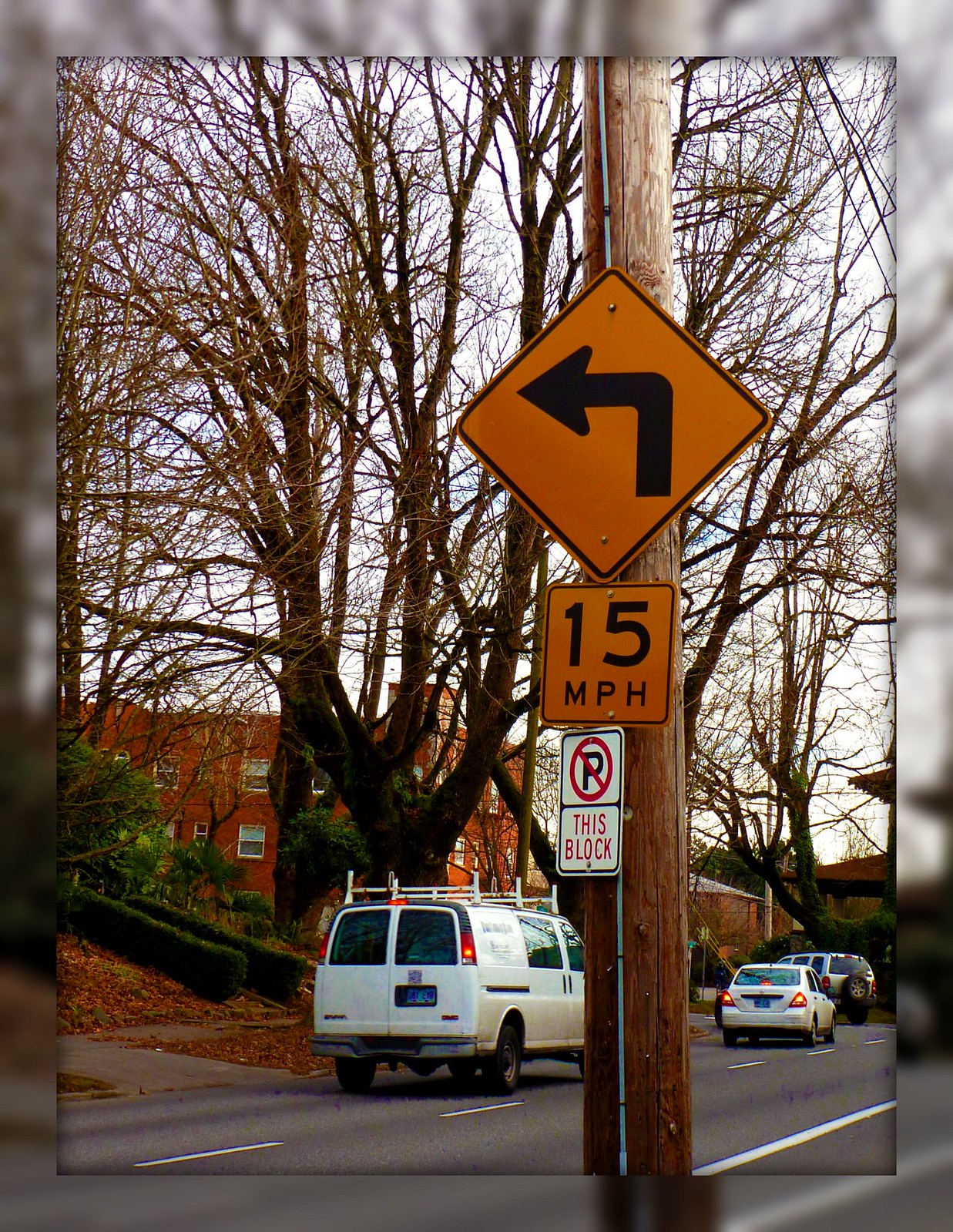A photograph taken in late fall captures a street scene, seemingly in America, possibly in New England or the Midwest. The light blue-gray sky lights up a row of three-story red brick buildings lining the opposite side of the street. Tall, bare trees and evergreen bushes, with some standing on sloped lawns, frame the left side of the scene. The ground is strewn with countless brown and orange fallen leaves.

Dominating the foreground is a wooden utility pole. It prominently displays an orange, diamond-shaped left turn arrow, below which is an orange sign indicating a speed limit of 15 miles per hour. Further down the pole is a white "No Parking This Block" sign featuring a red circle with a slash through a 'P'. 

Across the street, a white van with black tinted windows and heavy constructed racks is parked, with a white car in front of it seemingly making a left turn at the corner. Further down, a silver SUV is parked. The image carries a slight vignette effect with a drop shadow inset around the edges, adding a sense of depth to the photograph.